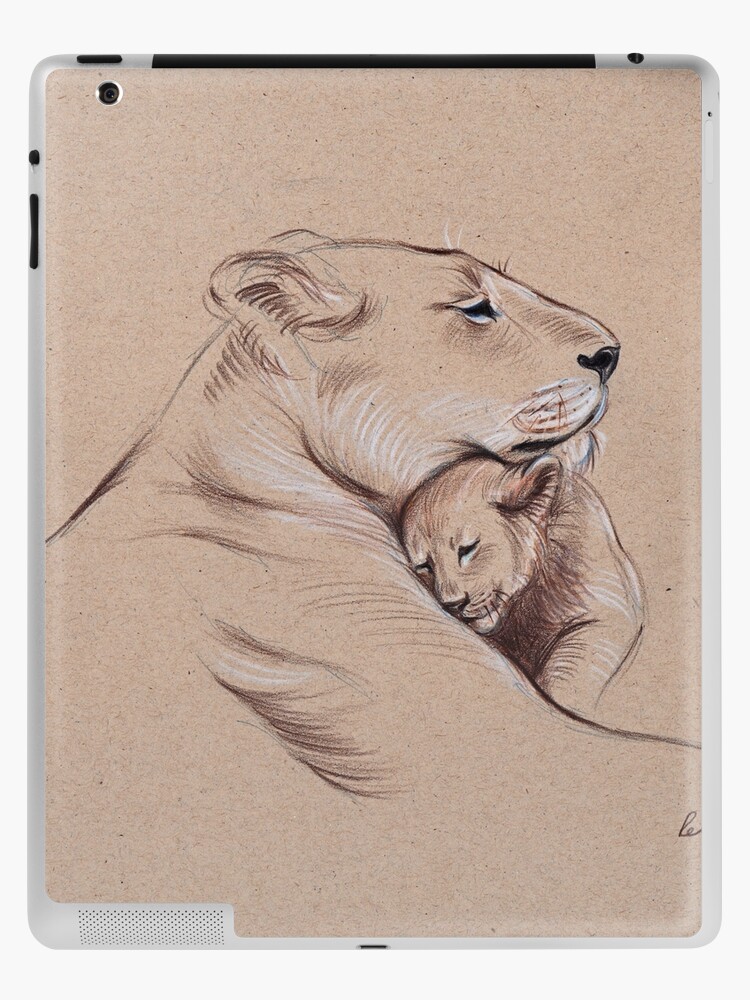The image features a detailed and professional drawing of a lioness and her cub set against a light brown background. The drawing, rendered in colored pencils of black, brown, and white, is displayed on the back plate of a metallic-framed tablet, identifiable by its camera on the top left, switch buttons on the left side, and a headphone jack at the top. In the drawing, the lioness, lying down with her head pointing to the right, has closed eyes, a black nose, and whiskers. The cub, snuggled comfortably under the lioness's head, also has closed eyes and a visible arm, contributing to the warm and relaxing atmosphere of the picture. The entire composition conveys a sense of serene connection between the mother and her offspring.